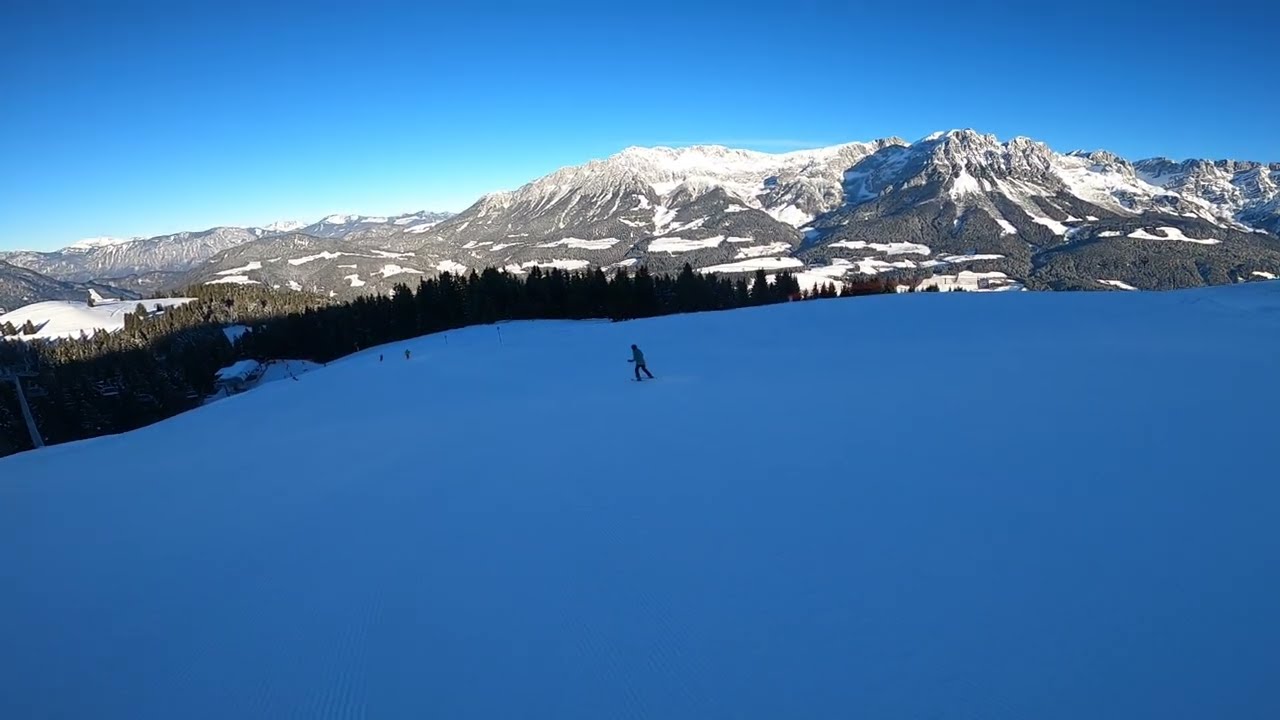In the photograph, a male skier is captured navigating down a snow trail at a ski resort. The skier is moving forward on a gentle slope framed by a landscape brimming with snow-capped mountains in the background. The horizon is dominated by an expansive mountain range, predominantly centered on the right side, with its peaks towering over the landscape. The mountains gradually descend towards the left, complemented by a series of lower plateaus and smaller mountain formations. 

In the distance, a few other skiers can be faintly discerned, though they are quite far away, with only two possibly identifiable. The extensive snow-covered terrain creates a serene, almost monochromatic scene, interrupted only by clusters of trees that appear in shades of dark black due to the shadows cast upon them. The snow itself has a light blue hue, likely reflecting the clear, bright sky above, which is a light blue with occasional patches of white and hints of darker shades creeping in. The overall ambiance of the photo evokes the pristine and tranquil beauty of a winter wonderland, with the solitary skier adding a dynamic element to the otherwise still landscape.